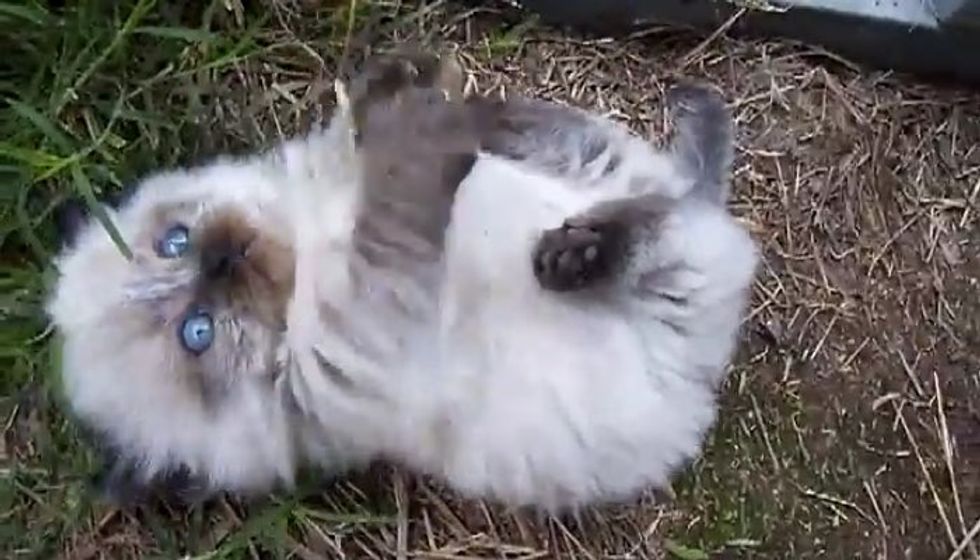The image depicts a charming, fluffy kitten lying playfully on the ground, its creamy white fur blending slightly into the background due to a soft blur or filter. The kitten, reminiscent of a Siamese with its bright blue eyes, dark gray ears, and similarly colored paws, sports a slightly chubbier, furrier appearance suggesting it’s a mix of another breed. The kitten's nose and tail tip also share the same dark gray hue. Positioned on its back, the kitten has its front paws endearingly raised in the air and its head nestled on a patch of grass interspersed with hay and moss, giving the scenery a rustic feel. In the top-right corner of the frame, a metallic object, possibly part of a table or chair, is partially visible, adding a touch of background detail to the cozy setting. Its playful posture and the light reflecting in its vivid blue eyes amplify the kitten's lively and healthy demeanor.